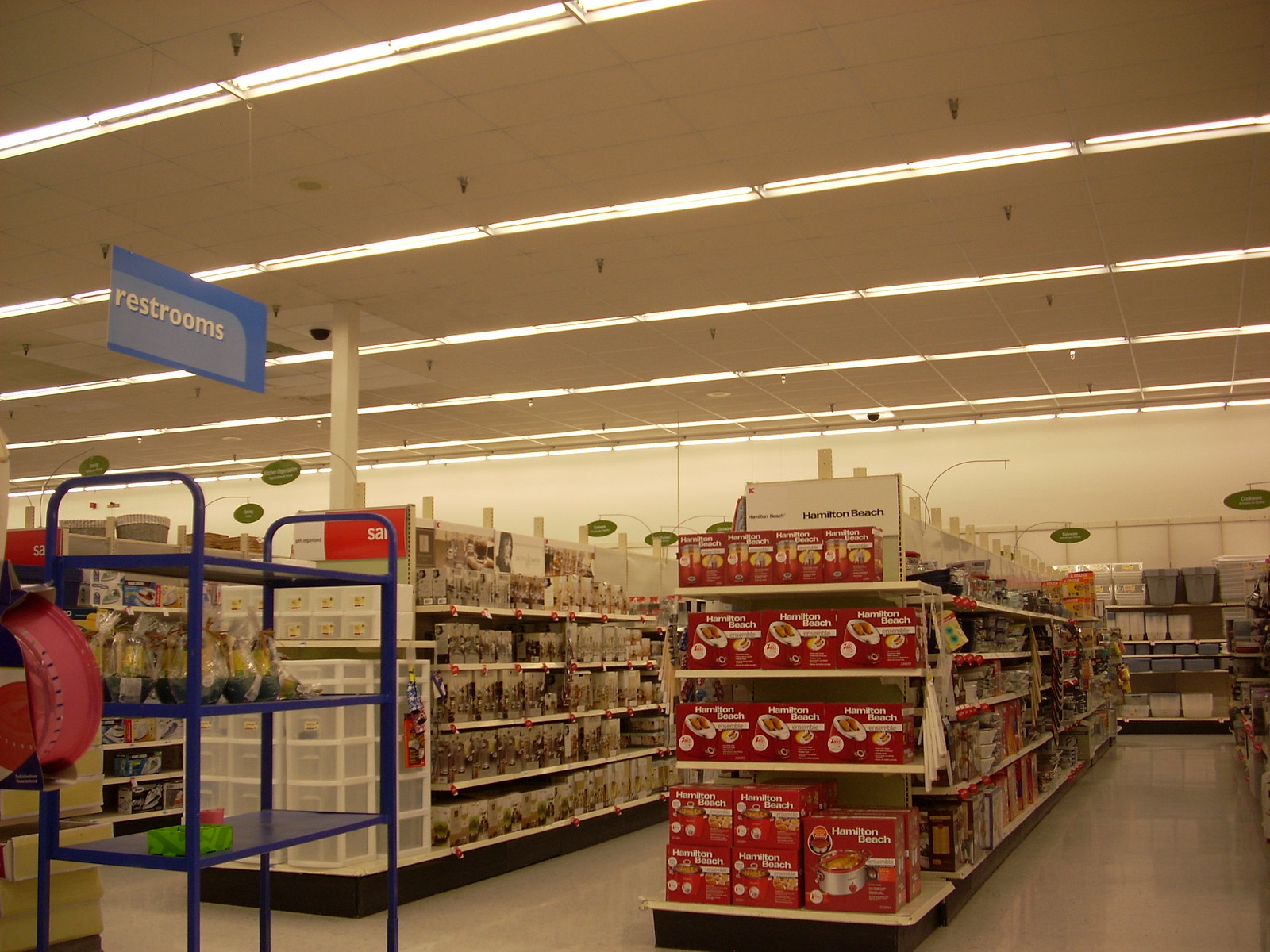In this detailed rectangular image of a supermarket, possibly Walmart, various items line the aisle shelves beneath fluorescent lights running diagonally from the upper right to the lower left. The photograph showcases multiple aisles filled with small home appliances, prominently featuring Hamilton Beach products, including kitchen gadgets like a hot appliance, a toaster, and a mixer. Among the merchandise, a blue cart stands in the foreground, likely used by a worker to move items around. Above, a blue sign with white lettering indicates the presence of nearby restrooms. The back wall is also stacked with products, completing the vibrant, bustling scene of this well-stocked store aisle.